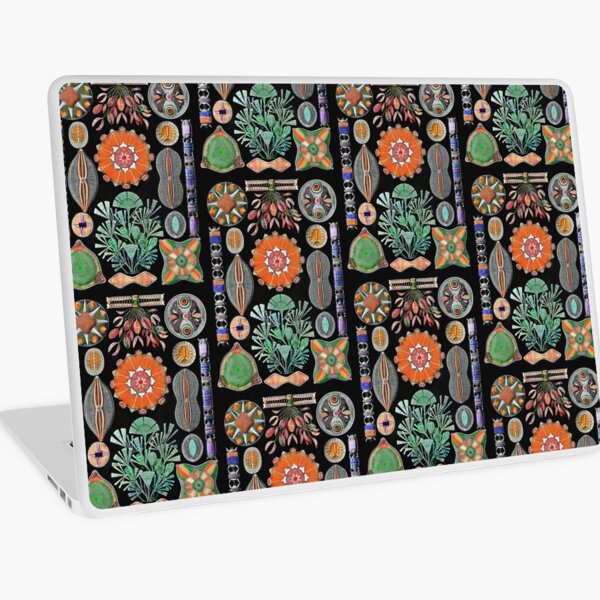The image shows the back of an Apple MacBook laptop, flat and white, with three visible ports of varying sizes on the side. The primary focus is the vibrant and detailed sticker or wrap covering the back of the screen, set against a pure white background. The design features a repeating array of colorful, gem-like shapes and organic patterns including an orange sun-like shape, green plant-like shapes with stems and fronds, and upside-down pink flowers. Additional elements include green circles with hourglass shapes, orange circles, blue peanut shapes with red stripes, and cat's eye marble shapes. These elements recur alongside blue lines, orange-dotted green circles with spikes, and eyeball-like shapes with red spikes, creating a visually striking and dynamic pattern across the laptop’s back.